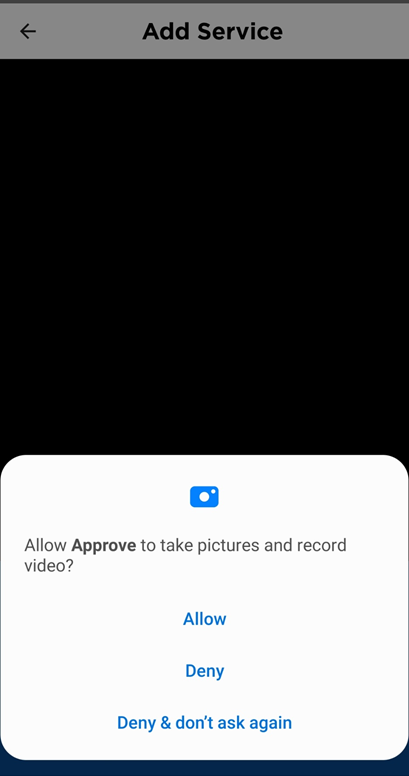This is an Android permission screen displaying a prompt for the app named "Approve" to gain access to the device's camera functionalities. 

The top header reads "Add Service." Below this header, there is a permission request card that occupies the bottom portion of the screen. The permission request asks, "Allow 'Approve' to take pictures and record video?" 

Three response options are provided: 
1. "Allow"
2. "Deny"
3. "Deny and Don't Ask Again"

The interface above the permission card is black, either obscured or intentionally left blank. The overall layout suggests the device might be in light mode, although it is not definitively clear. This concise yet informative screen is designed to ensure users make an informed decision about granting camera access to the "Approve" app.